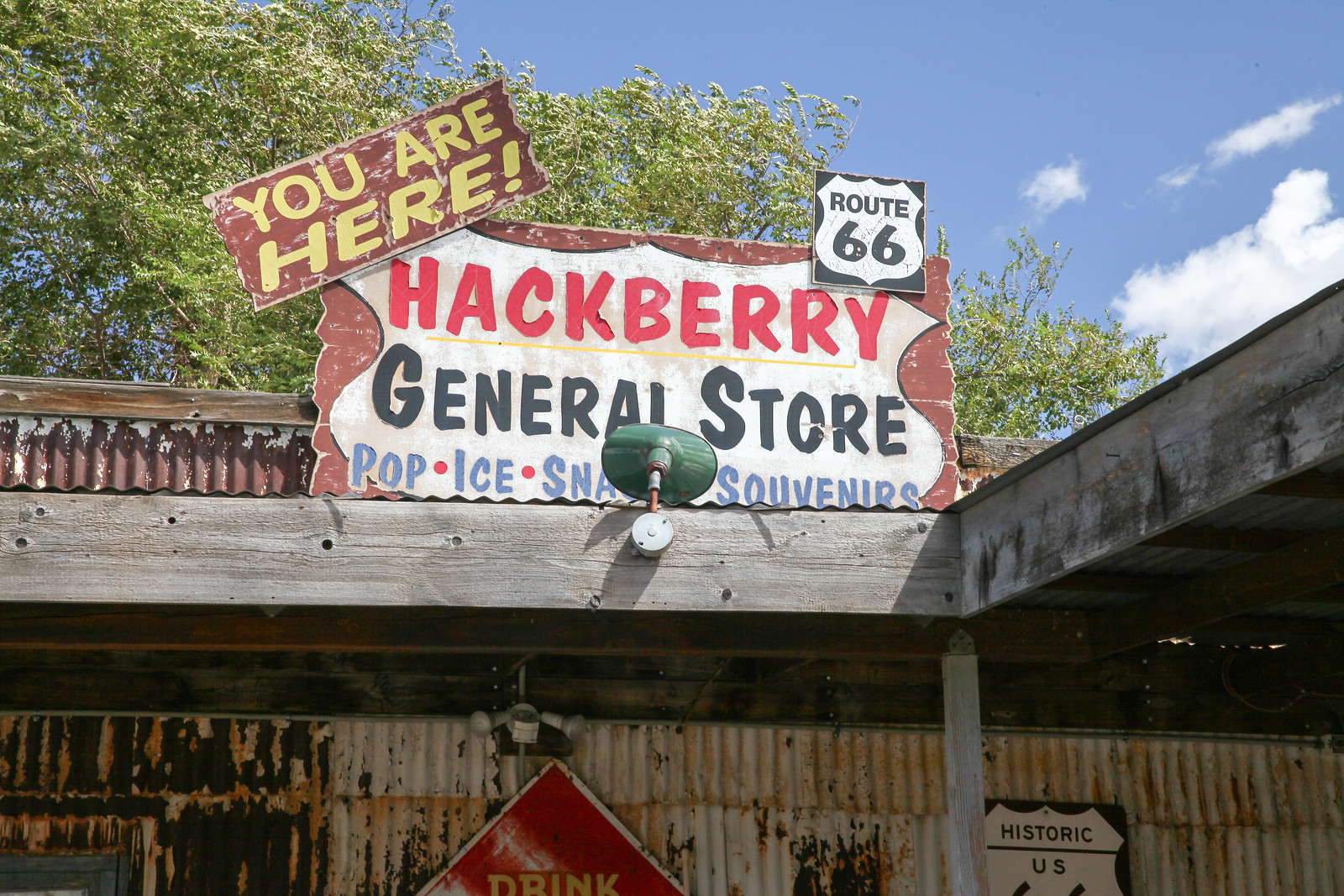The photograph, taken outdoors on a sunny day, captures a timeworn facade of the Hackberry General Store along Route 66. The upper right corner of the image reveals a clear blue sky with a few scattered clouds, while the top left and center of the frame show green leaves on trees, hinting at a lush environment. Dominating the center is a very beat-up, old-fashioned sign, mounted on a wooden frame. The sign, with its colors largely scratched and faded, prominently reads: "You are here, Route 66, Hackberry General Store, Pop, Ice, Snacks, Souvenirs". Atop this sign is a vintage outdoor light, presumably meant to illuminate it at night.

The store itself appears to be constructed from corrugated metal, adding to its rustic, abandoned feel. Below the main sign, partially visible, is a red, diamond-shaped logo that says "Drink" in faint yellow lettering. To the right of this, there's a historic road sign that reads "Historic U.S. 66". The overall aesthetic suggests a place steeped in history but long past its heyday, evoking the iconic allure of America's famous Route 66.